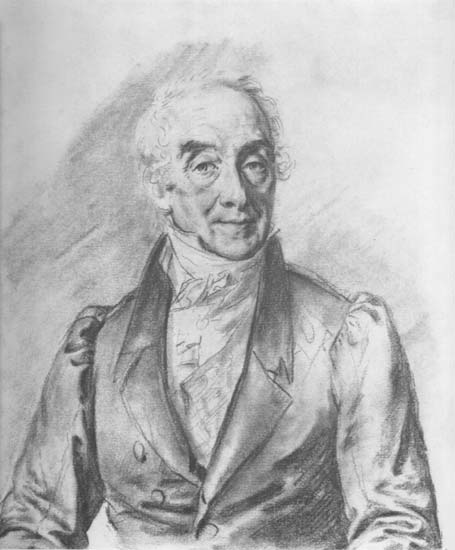This monochrome artist's rendering is a detailed indoor portrait of a distinguished, elderly white gentleman, sketched in a classic style suggestive of the 19th century. The man, who appears to be in his 60s, exudes a serious yet slightly stern demeanor. He is characterized by his balding head with wispy hair on the sides and a high forehead. His large nose and piercing eyes, which gaze slightly away from the camera, add to his distinguished visage. He's garbed in a historically styled dark jacket, buttoned along the left side beneath an upturned collared white shirt. The jacket's sleeves appear slightly bulky, hinting at layers of clothing beneath. He is not wearing a tie, and his high shoulders add to his dignified presence. The backdrop is a gradient of gray with darker splashes around his head, enhancing the depth of this finely detailed black-and-white illustration. His hands rest in front of him, suggesting a seated pose, though only the upper part of his body is visible. The paper itself is an off-white color, completing this evocative sketch of a refined gentleman from a bygone era.